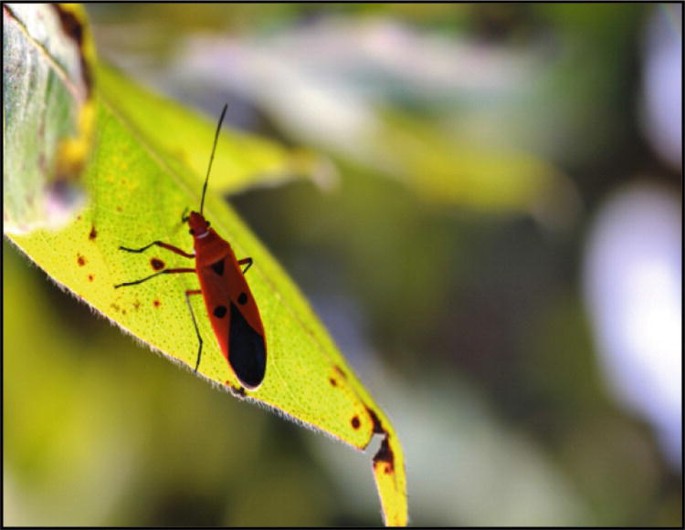In this close-up, color photograph of a beetle on a leaf, the subject is intricately detailed. The beetle, predominantly orange with distinctive black markings, is positioned on the left side of the image, its head facing the top left corner. It features a black triangle on its upper body near the shoulders, two black dots midway down its back, and a black teardrop shape near the tail. The beetle's segmented legs are visible, with three legs on the left side and one on the right, and its antennae extend from its head, one barely visible and the other sticking straight out.

The beetle is perched on a light green leaf, speckled with brown spots, prominently angling diagonally from the top left toward the bottom center of the image. A second, out-of-focus leaf forms a sideways V in the background, pointing away from the viewer. This leaf, as well as the rest of the blurred dark green shapes in the background, provides a contrasting backdrop that highlights the intricate details and vivid colors of the beetle and its foreground leaf. The landscape-oriented photograph captures the scene with a high level of realism, drawing attention to the delicate details of nature.